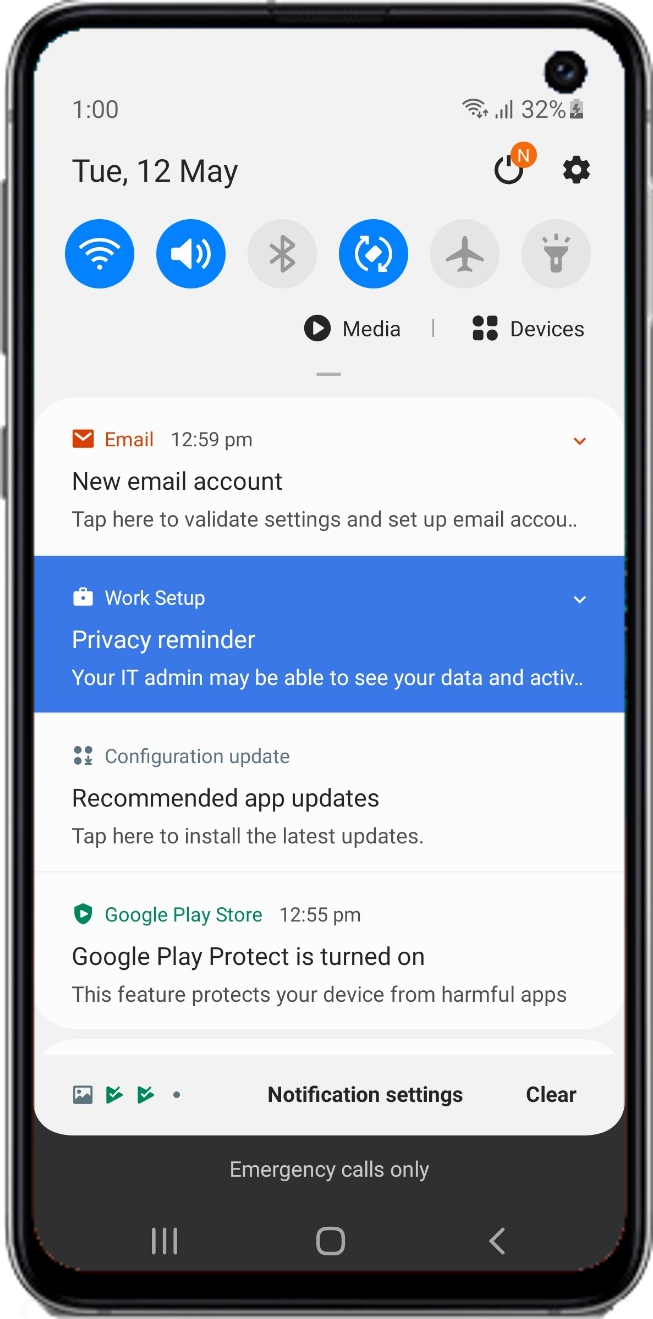**Caption:**

A three-dimensional light silver cellphone is displayed against a stark white background. The device features buttons on its left side and a power button with an orange circle housing a white "N" on the upper right. The screen shows a status bar at the top left corner indicating "1 and 1," with Wi-Fi and cellular signal bars, and a 32% battery icon on the right. It's Tuesday, 12 May, as mentioned just below the status bar. 

On the right, below the Wi-Fi and battery indicators, is a settings icon. The quick settings panel displays icons for Wi-Fi, sound, Bluetooth, screen rotation, and airplane mode. Wi-Fi, sound, and screen rotation icons are highlighted in blue, while the rest are gray. 

Underneath the settings icons, "Media and devices" is labeled. Further down, at 12:59 p.m., a notification prompts the user to set up an email account: "New email account tap here to validate settings and set up an email account." Below this, a blue strip with white text states, "Work setup privacy reminder: your IT admin may be able to see your data and activity." The bottom of the screen reverts back to a white background with the text, "Configuration update."